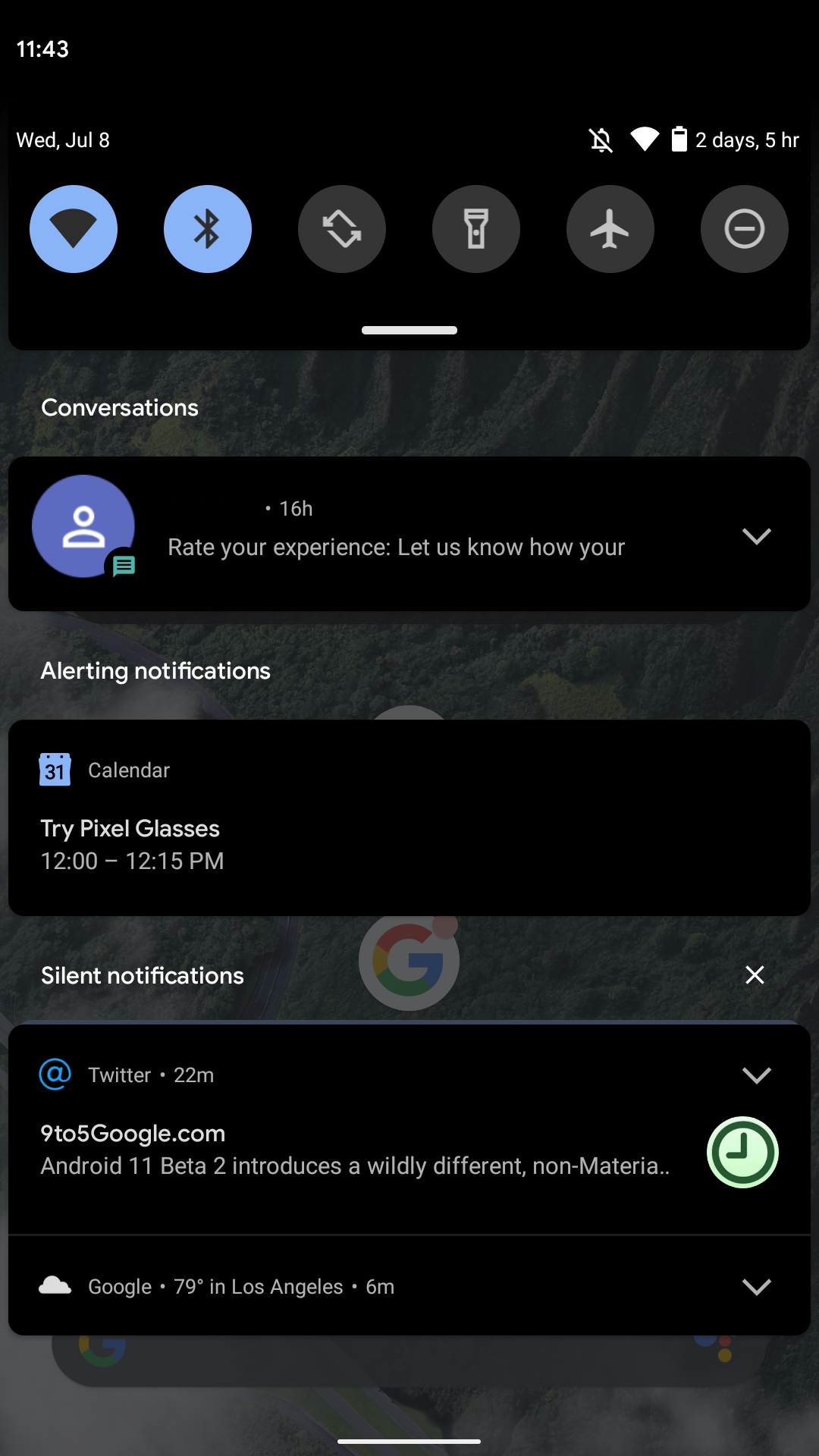A screenshot displays a Google cell phone screen featuring the quick menu in night mode with a black background. At the top of the screen, there is a horizontal row of circular icons. The first icon on the far left is the Wi-Fi icon, active and highlighted in blue. Next to it, also active and in blue, is the Bluetooth icon. The subsequent icons from left to right are the flashlight icon, the airplane mode icon, and the minimize window icon, all remaining mostly unhighlighted.

Beneath this row of icons, a white bar labeled "Conversations" appears in small white font in the top left corner. Below this label is a visible text message. Descending further, another white font label reads "Alerting notifications," followed by a box containing a calendar notification. Toward the lower left section of the screen, the label "Silent notifications" appears in small white font, beneath which there is a Twitter notification.